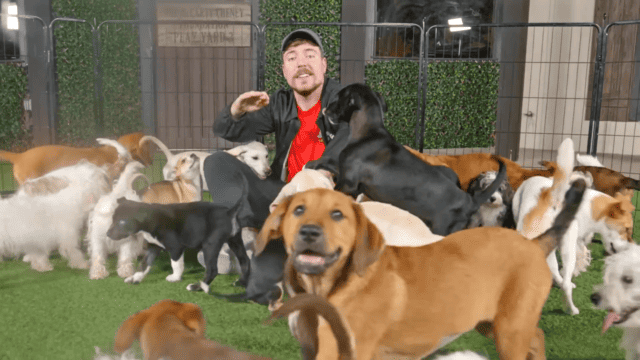In the image, a bearded man is sitting or kneeling in the center of a fenced-in kennel area, surrounded by an assortment of at least 15 to 20 dogs of various breeds, sizes, and colors. He is attired in a gray baseball cap, a black jacket over an orange t-shirt, and he has his right hand raised, possibly to pet one of the dogs. The green ground, which appears to be either grass or turf, is barely visible due to the sheer number of dogs. There is a prominent brown dog with a black tail in front of him, looking towards the camera with its mouth open. Another black dog is seen jumping onto his legs, and numerous other dogs of black, white, and mixed colors are scattered around him. In the background, a black metal fence encloses the area, which appears to be a dog training or kennel zone, with a building featuring a green wall and a door visible behind the fence. The man is smiling and looking directly at the camera, seemingly at ease amidst the lively scene of playful dogs.